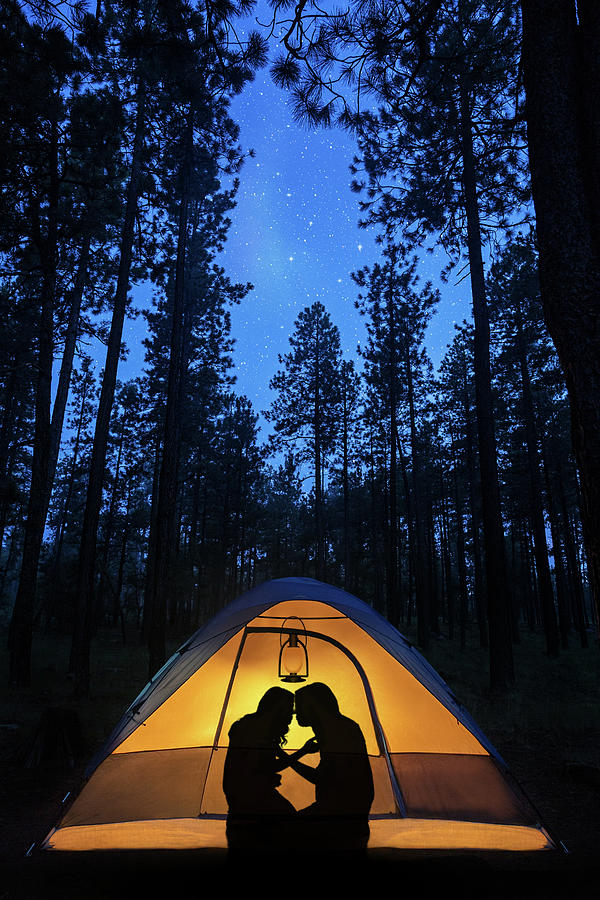The image depicts a serene twilight scene featuring a small, dome-shaped tent nestled in a forest of towering pine trees. The deep blue sky, speckled with stars, suggests it is evening, and there is just enough light to outline these majestic trees. Inside the tent, illuminated by a warm orange glow from a hanging lantern, the silhouettes of a man and a woman can be seen kneeling and embracing tenderly, as if about to kiss. The tent's rounded triangular shape and its snug, intimate lighting create a cozy and romantic atmosphere amid the tranquil wilderness.